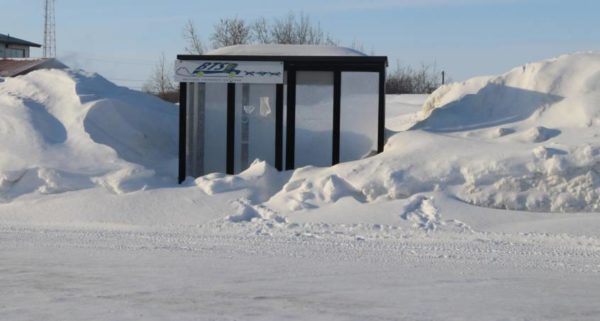In a snowy winter landscape, a clear, sunny day illuminates a solitary bus stop standing beside a road, almost buried under mounds of snow. The bus stop, constructed from metal and glass with black-framed rectangular panels, has a slightly rounded roof lightly covered in snow. A sign marked "BTS" hangs on the front of the bus stop. Footprints trace a path through the snow to the bus stop, which is surrounded by large piles of snow, likely cleared from the road. Off to the left, there's a glimpse of a house's roof and a metal communication tower. In the background, the tops of some bare trees stretch out, further defining this serene winter scene. The sky is a wispy blue with streaks of white clouds, adding to the overall brightness that makes the snow glisten. Despite the inviting structure, the bus stop appears inaccessible due to the heavy accumulation of snow around it.